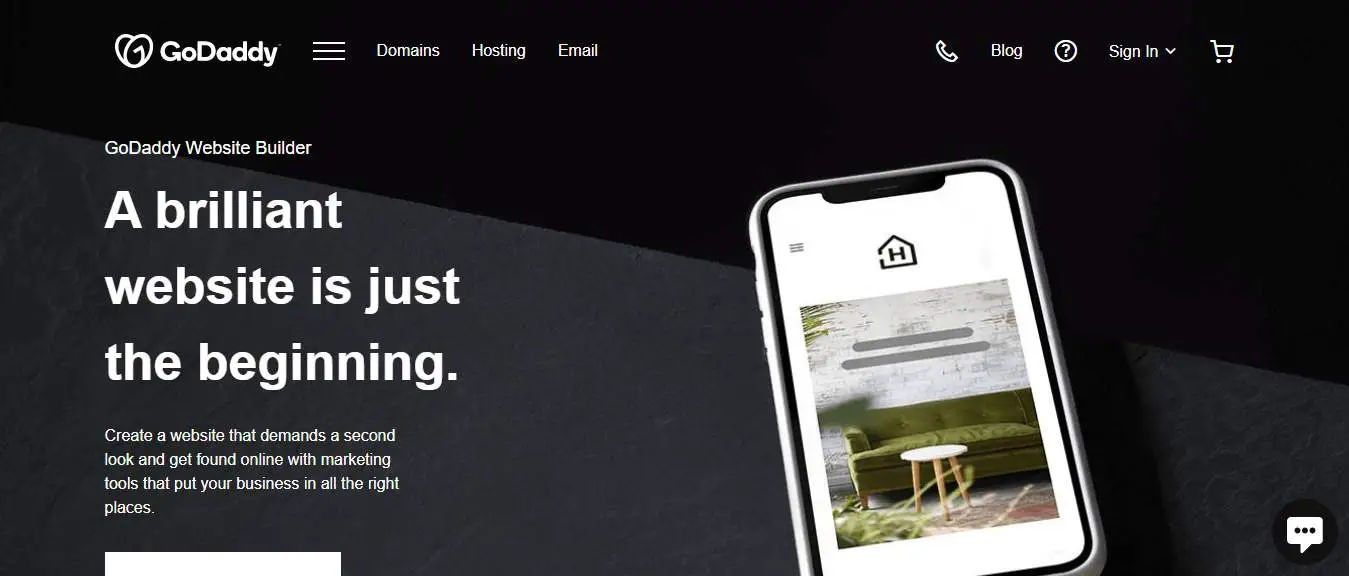This is a detailed screenshot of the GoDaddy.com homepage. The main section of the screen features a bold, white text stating, "A brilliant website is just the beginning," set against a black background. Beneath this text, there's an image of a mobile phone, emphasizing the website's mobile-friendly capabilities. 

At the top of the screen, the navigation bar contains several submenus, including "Domains," "Hosting," and "Email." To the right of these options, there is a phone icon for contacting GoDaddy support. Next to the phone icon are links labeled "Blog" and a question mark symbol for help or FAQs. Additionally, there is a sign-in toggle for existing users, followed by a shopping cart icon. 

This screenshot captures the essence of GoDaddy.com, showcasing its various services like purchasing domains and setting up websites or apps.